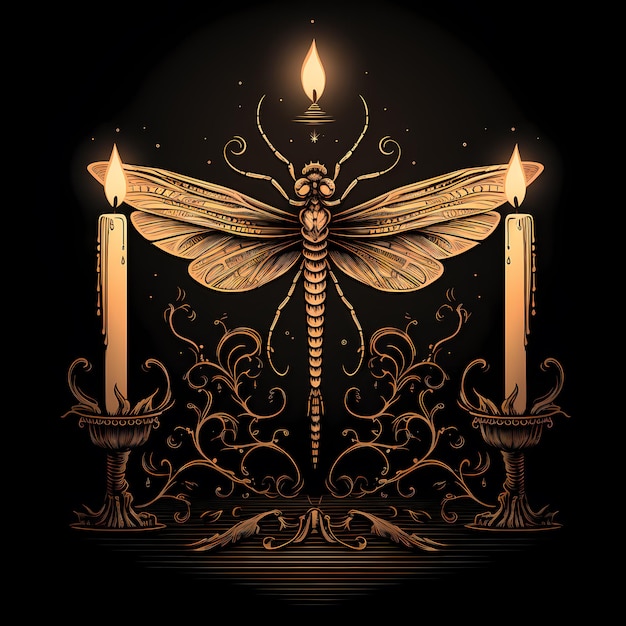This detailed artwork features a majestic, gold-hued dragonfly, prominently displayed against a deep black background. The dragonfly stands upright, balanced on the tip of its tail, with elegantly fanned-out wings that frame two tall, lit candles positioned at either end. Above its head, a third candle flickers, enhancing the ethereal quality of the scene. The intricate dragonfly, with its curly antennae and legs, appears almost metallic, reflecting shades of brass, gold, dark brown, and hints of blue where the candlelight illuminates its body.

Beneath the dragonfly is an ornate candle holder, adorned with intricate, curly patterns resembling a fleur-de-lis design, in complementary shades of brass and yellow. The artwork's background is adorned with twinkling white stars, adding a magical touch. The candles, with their drippings visible, cast a warm light that imbues the composition with an enchanting, luminescent glow, suggesting the piece could be an elaborate lamp or lantern.

The dragonfly's wings are impeccably detailed, with numerous lines creating intricate shapes and structures, echoing the overall ornate and surreal aesthetic of this captivating piece.